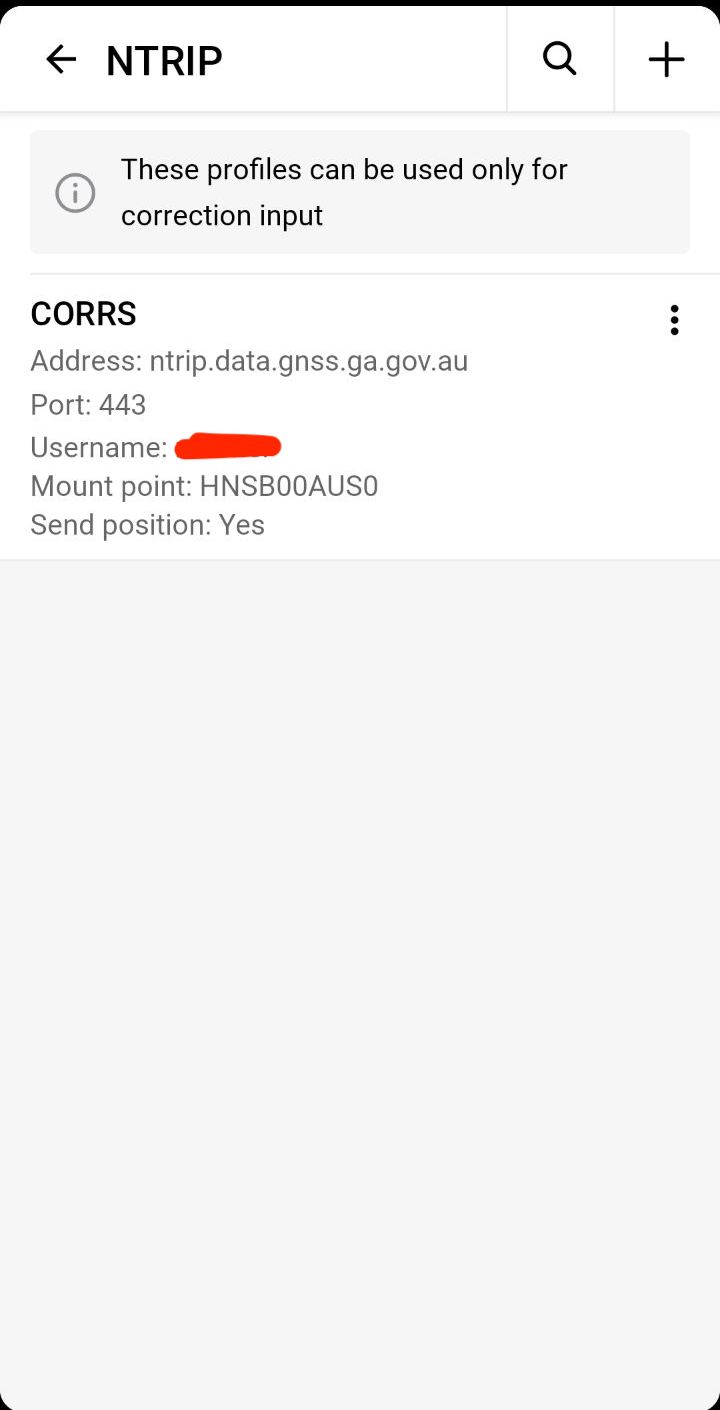The screenshot, taken on a smartphone, displays an application called "nTRIP." At the top of the screen, there's a navigation bar with a back arrow, followed by the title "NTRIP" in all capital letters. To the right of the title, there is a magnifying glass icon for the search function, a plus sign button, a thin divider line, and an information icon represented by a gray lowercase 'i' inside a gray circle.

Below the navigation bar, the text reads, "These profiles can be used only for a correction input," followed by the label "CORS" in bold, black capital letters. To the right of this text, there is a vertical three-dot menu option. 

The section below contains several lines of grey text detailing the input settings:
- Address: ntrip.data.gnss.ga.gov.au
- Port: 443
- Username: [Redacted with red slashes]
- Mount Point: HNSB00AUS0 (in all caps)
- Same Position: ES

The background is predominantly white, with a black line at the top featuring slightly curved areas that reveal the white background beneath. At the bottom of the image, there is a small portion of black with curved edges meeting sharp corners, consistent with typical smartphone screen design elements.